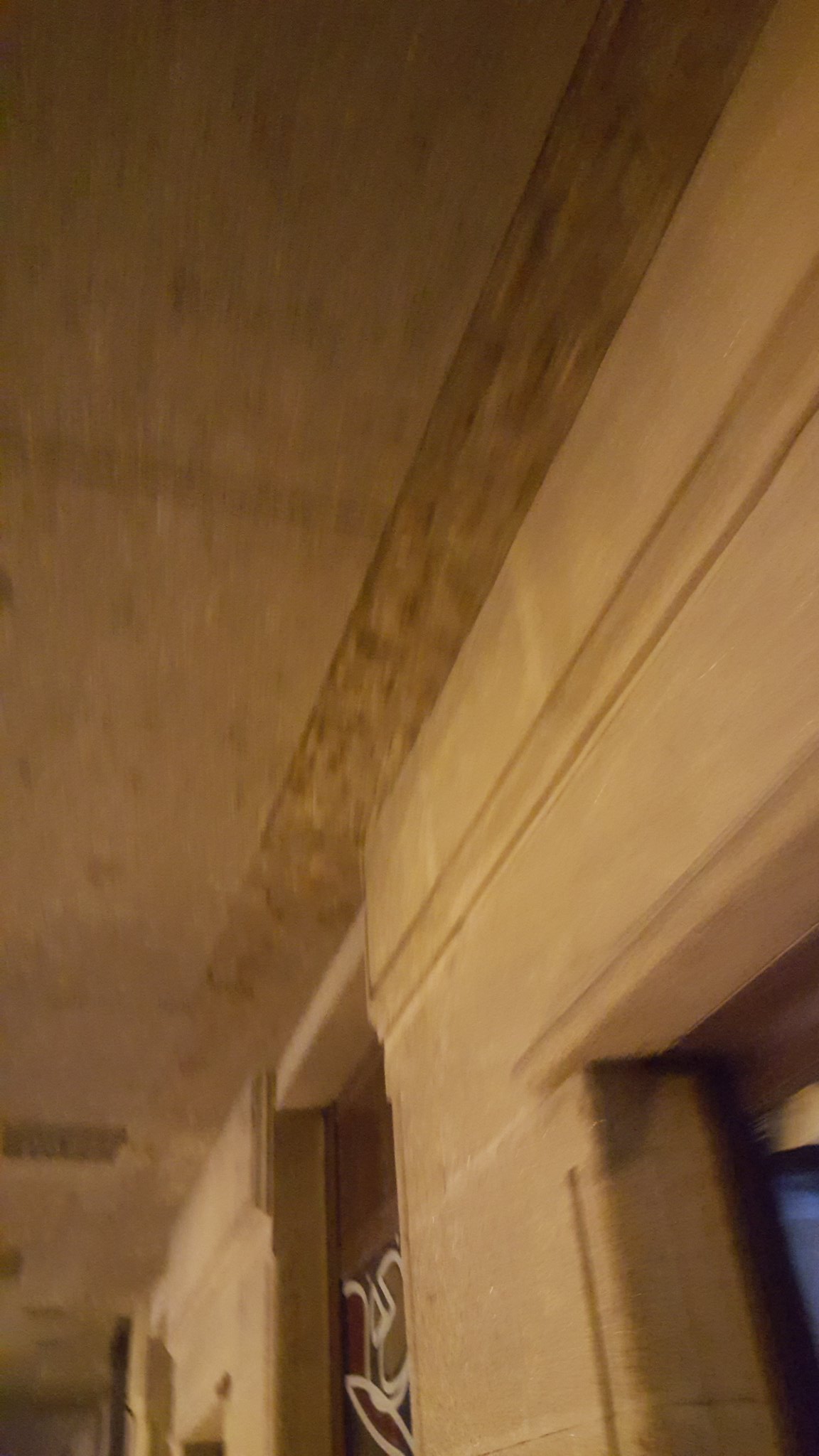The image depicts the ceiling and upper section of a stone corridor infused with a predominantly pale, tannish color scheme. The ceiling is mottled with light and dark brown sections, particularly darker near the right side where it meets the wall. A vent is visible in the bottom left of the ceiling, and the corridor seems to extend into the distance in this direction. To the bottom right, there's a doorway that slightly reveals white elements possibly resembling stickers or decals. The corridor's wall, matching the tan hue of the ceiling's center, features a border along the top edge, and a wooden recess with white lines is noticeable towards the bottom. The setting conveys a structured, possibly aged architectural space with elements like vents and repeated patterns in the ceiling, enhancing its intricate design.